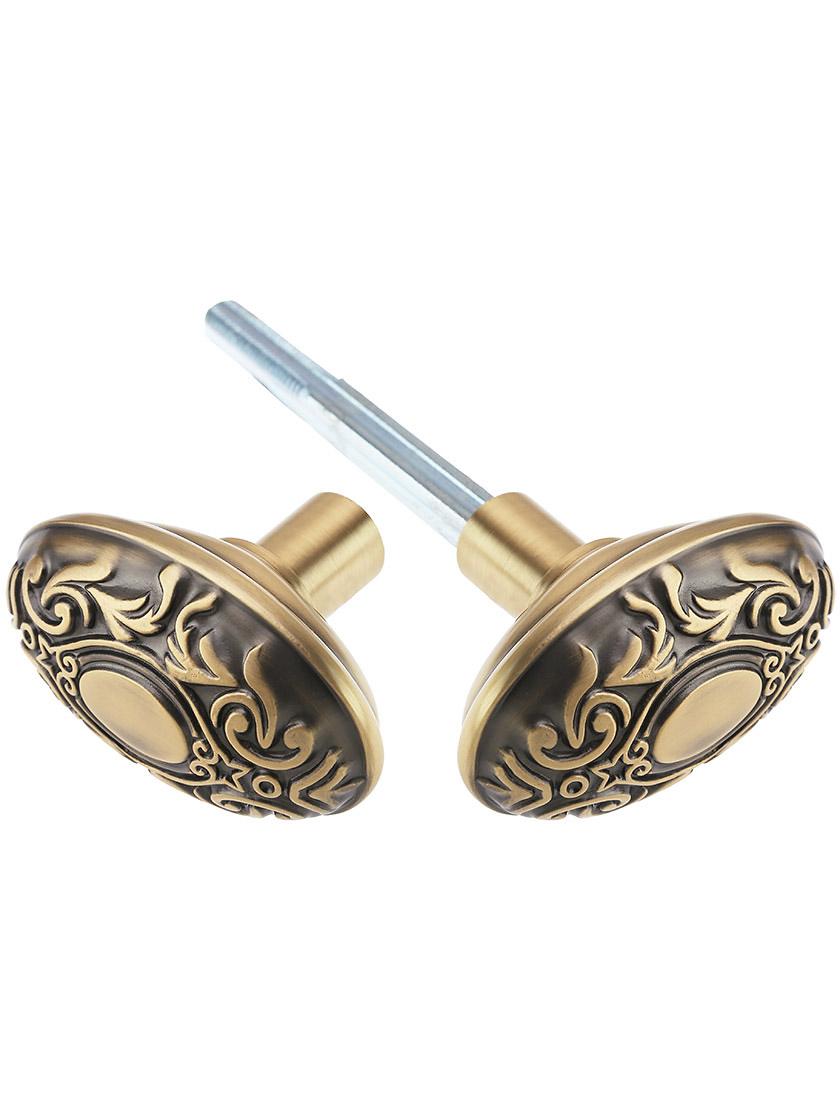In this highly detailed, up-close photo set against a pure white background, two identical rounded objects are prominently displayed. These objects are small and intricate, resembling vintage cufflinks or possibly stud earrings due to their delicate size and design. Each piece features a circular face with a gold and brass-toned finish, adorned with elaborate engravings. The detailed design includes a central circle surrounded by fleur-de-lis motifs, complemented by a couple of stars and possibly leaf-like or wind-inspired embellishments. One of the objects has a metal rod extending from it, suggesting its functional purpose, which might be to insert through a shirt cuff or to secure an earring. The objects are positioned side by side, slightly diagonal to each other, forming an X-like orientation, adding a dynamic aspect to the composition of the photograph.